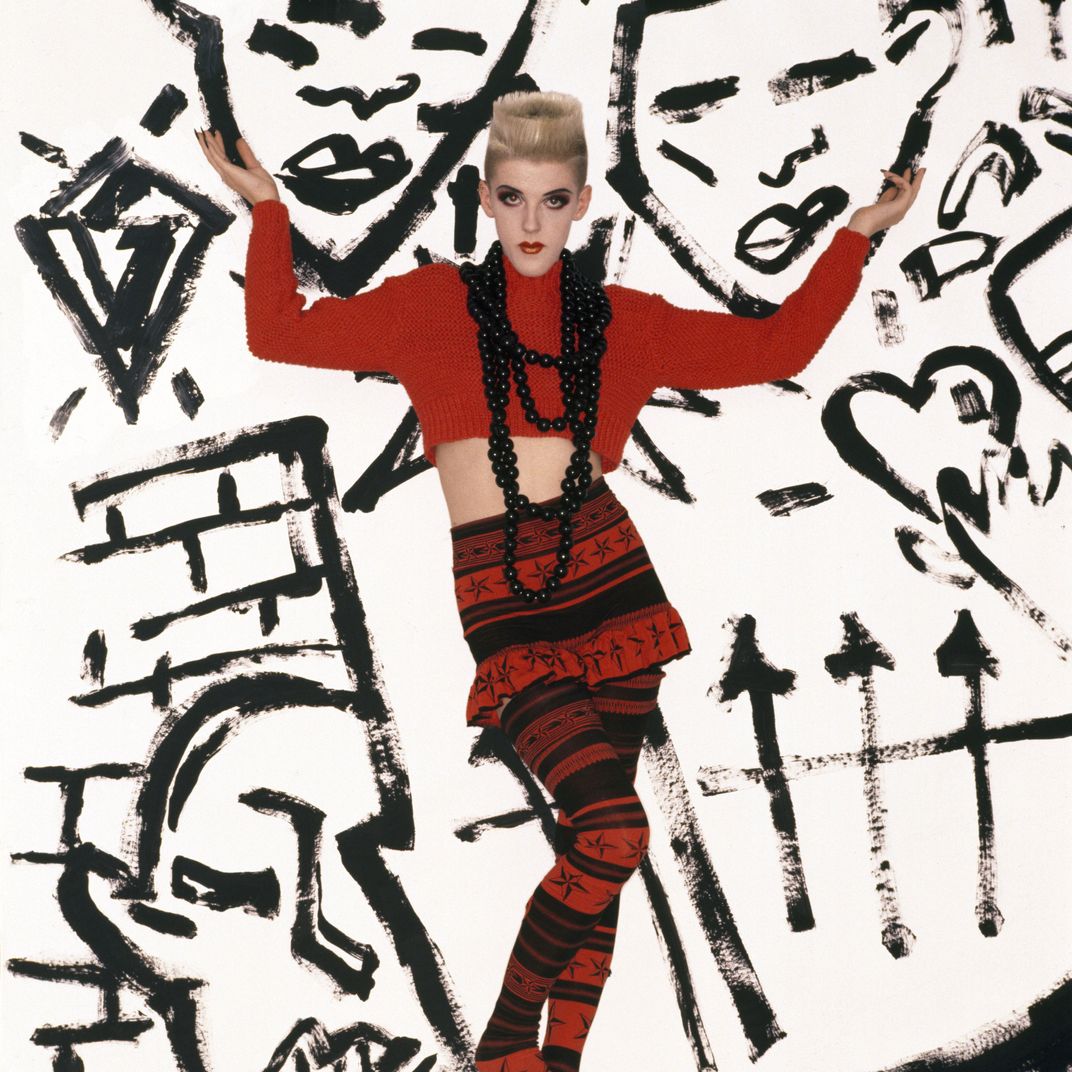The image prominently features a striking figure posing dynamically against a white background covered with graffiti-like black markings, resembling child-like scribbles that include various elements such as faces, a fence, a wall, a diamond, arrows, and a heart. The individual, possibly a model or an artist, has a tall crew cut hairstyle reminiscent of Vanilla Ice, with dark eye makeup and noticeable red lipstick. They are dressed in a red knitted crop top exposing the midriff, accessorized with a large black beaded necklace. Completing the outfit is a red and black striped skirt matched with leggings or socks, creating a cohesive and edgy ensemble. The pose is expressive, with arms extended to the sides and legs crossed, almost as if in mid-dance.